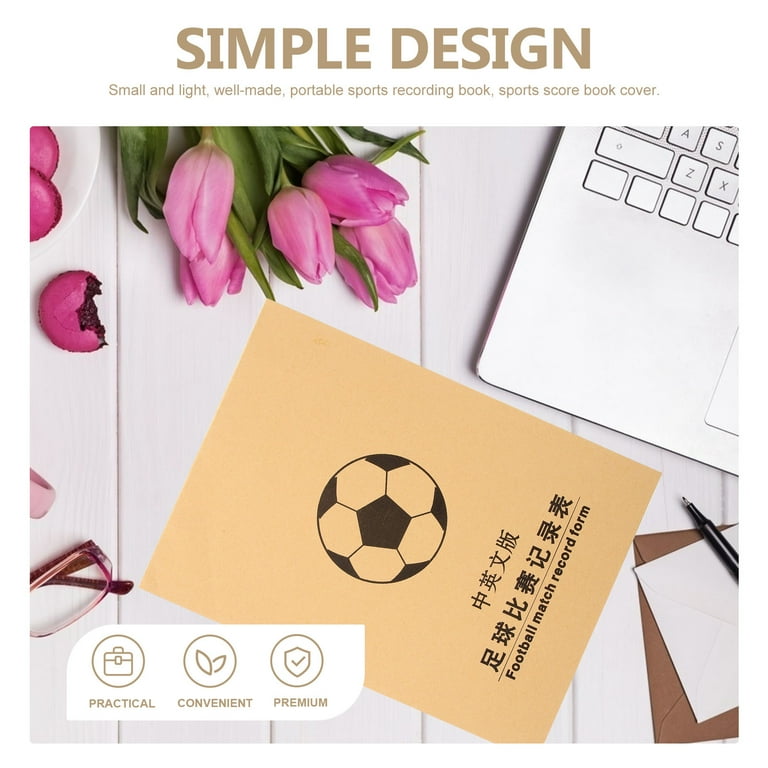The image, likely an advertisement, showcases a minimalist and well-designed sports recording book on a white wooden desk surface. At the top in bold brown letters, it reads "Simple Design," with the smaller text below stating, "Small and light, well-made, portable sports recording book, sports scorebook cover." The focal point of the image is a yellow pamphlet, adorned with a drawing of a soccer ball and Japanese characters, labeled "Football Match Record Form." Surrounding the pamphlet, in the top right corner, partly visible, is a laptop keyboard. The top left corner features a bouquet of pink tulips. The bottom left corner displays eyeglasses, an envelope, and a black pen. The bottom of the pamphlet includes three icons labeled "Practical," "Convenient," and "Premium."